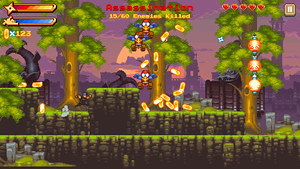The image is a captivating screenshot from a side-scrolling platformer video game set in a lush forest environment. The scene showcases a series of grassy, tufted platforms where the player's character is actively running and jumping. Menacing the character are three enemies, all airborne in mid-jump, adding to the intensity of the moment. A distinct blue bird with a yellow beak, dressed in what appears to be a reddish pilot bomber's uniform, is visible at the top of the screen. This bird is dropping yellow-orange pills or canisters that seem to be explosive in nature, adding an element of danger. A shuriken is also prominently seen flying through the air, suggesting that the character might be equipped with ninja-like abilities. At the top of the screen, red text reads "Assassination," indicating a nearly completed objective with "15 out of 16 enemies killed." This dynamic scene is filled with action and tension, highlighting the game's challenging and engaging gameplay mechanics.